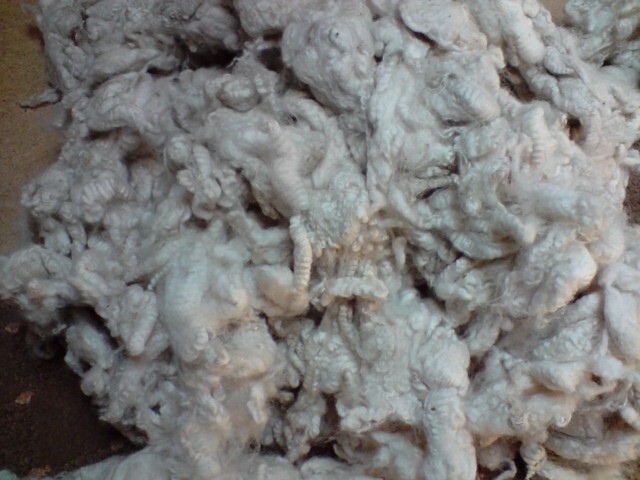In this detailed image, we observe a large pile of white material, predominantly filling the frame with varying textures and shapes. The lower left corner reveals a brown background, possibly a table or counter, with a small patch of dirt. This backdrop extends towards the upper left, transitioning into a beige wooden color. The material itself appears to be shorn sheep's wool, showcasing an array of forms—some sections are bright white and fluffy, resembling cottony insulation or meticulously pulled yarn, while other parts are darker and tightly woven, akin to dreadlocks. Certain areas look dense and blob-like, with signs of possibly having been wet, giving it a droopy, heavy appearance. The lighting in the image is uneven, highlighting one side of the pile brighter than the other, which could result from room lighting or natural light streaming into this cutting area.